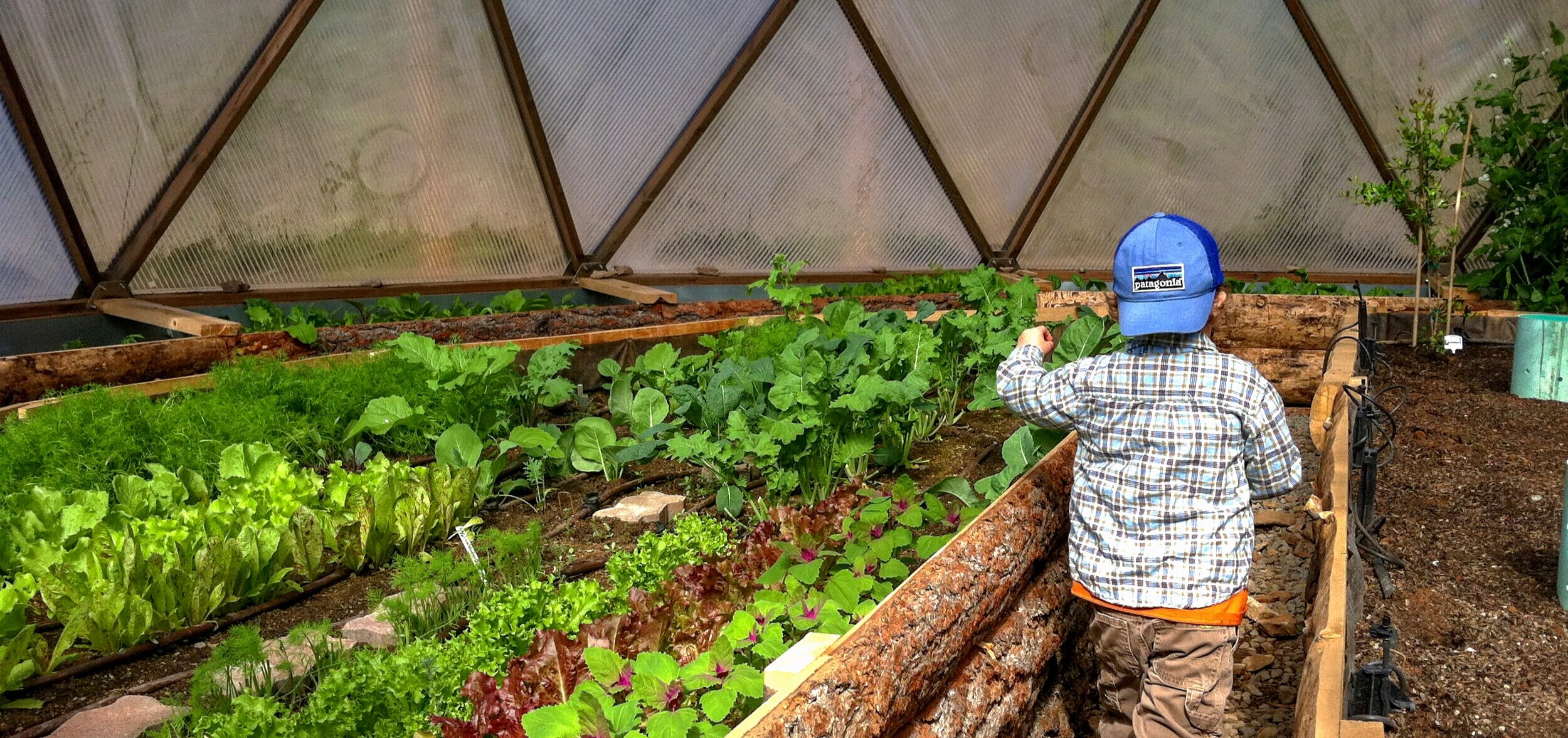The image is a detailed, color photograph capturing a young boy walking inside a greenhouse. The boy is facing away from the camera and sports a backwards blue baseball cap, a plaid long-sleeved button-down shirt in shades of white and dark blue over an orange shirt, and brown cargo pants. To the left of the boy, there is a prominent raised garden bed lined with what appear to be pieces of hand-cut logs, filled with various rows of green plants and vegetables, including turnips. The right side of the image shows bare dirt leading to another raised bed. The background reveals the triangular, V-shaped support beams of the greenhouse, which is covered with either semi-transparent fabric or glass panes, enclosing the entire area in a bright but sheltered environment. Green plants flourish near the left side of the frame against this unique structure, completing the serene garden scene.